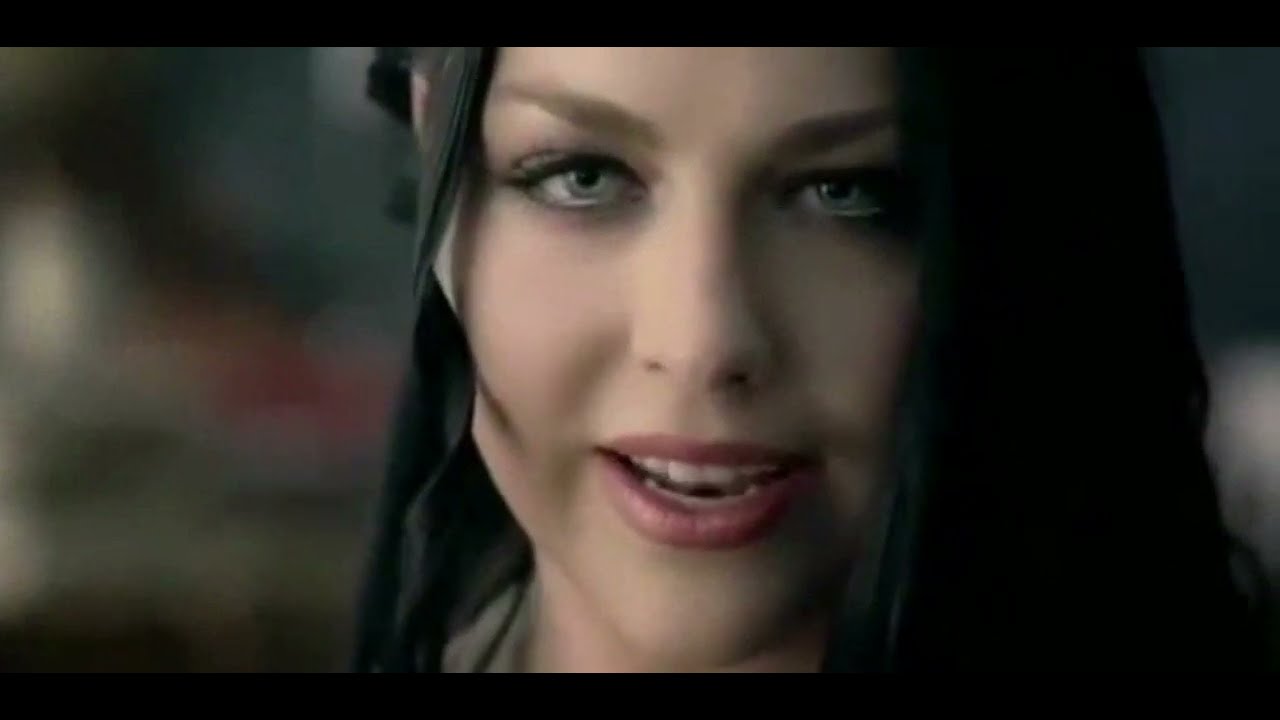The image features a close-up of a young, white woman in her 20s with dark black hair, wavy and possibly curled in sections, softly framing her face. Only her face is visible from just above her forehead to her chin, with the background heavily blurred out, leaving her features as the focal point. She has striking light hazel eyes that have a hint of light blue, accentuated with mascara. Her slightly parted lips reveal a light pink lipstick, and she appears to be in the middle of mouthing a word or mid-sentence, which gives her expression an engaging, almost animated quality. Her eyebrows are somewhat faded, and a couple of turquoise hair strands rest over her left cheek, adding a unique touch to her overall appearance. The lighting and makeup highlight her clear skin, and the image is so close that finer details of her attire or surroundings are indistinguishable. She exudes a youthful, expressive charm, reminiscent of a performer or someone in a casually poised moment.